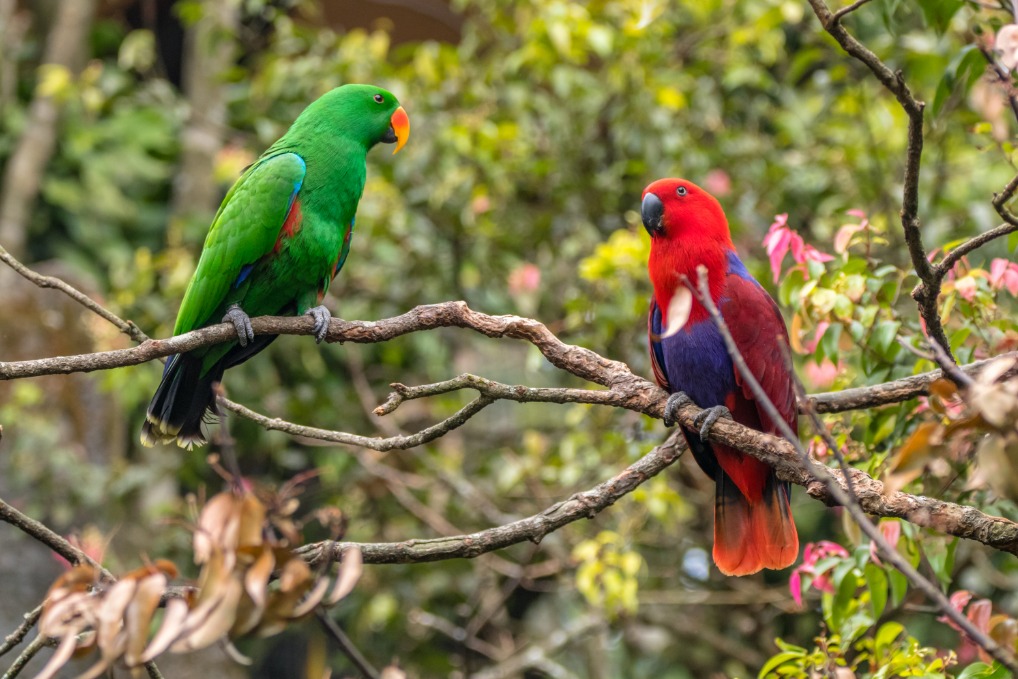The image captures a vibrant daytime scene of two parrots perched on a tree limb amidst a lush, green forest backdrop. The left parrot is a Mulliken Eclectus with striking green plumage, an orange beak, and blue accents on its wings, while the right parrot, likely an Amazon parrot, boasts a vivid red head, purple belly, maroon wings, and an orange tail, highlighted by a black beak. The background is beautifully blurred with a bokeh effect, bringing the birds sharply into focus. Both parrots appear to be engaged in a mutual gaze, illuminated by natural sunlight filtering through the foliage, creating a clear, colorful, and detailed composition.